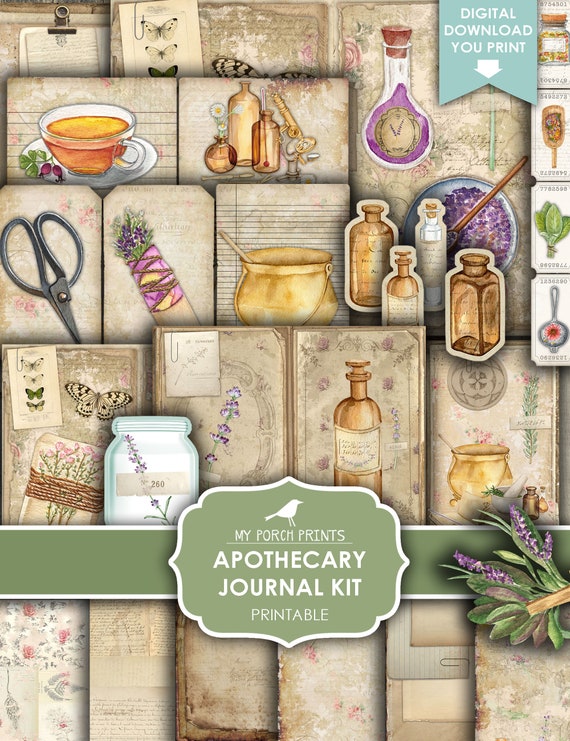This image is a detailed promotional piece advertising a digital download titled "Apothecary Journal Kit," created by My Porch Prince, whose logo features a white bird. This printable artwork has a vintage, artisanal feel, displaying a collection of apothecary items like old medicine bottles, jars, scissors, and other traditional pharmaceutical objects, set against a faint gray background with minimalistic designs and floral patterns. Central visual elements include a soothing bundle of lavender, a teacup, butterflies, a clipboard, a potion bottle, and a bowl of fruit, all sketched in an intricately detailed style. The upper right corner of the image clearly states the downloadable nature of the product with the label "Digital Download Uprint." This aesthetic and nostalgic print would make a charming addition to a bathroom, either as a framed piece or even used as wallpaper.